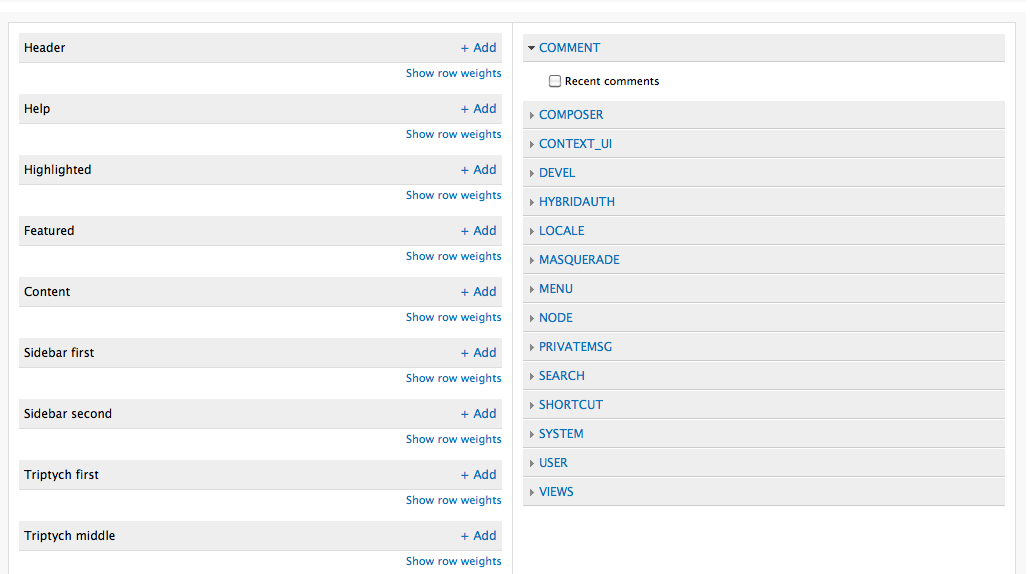This landscape-oriented screenshot depicts a structured, two-column form layout. The upper left-hand corner features a prominent header. To the right of the header, there is a blue "Add +" button followed by a line reading "Show row weights."

In the left-hand column, there are nine rows, each similarly formatted with an "Add +" button at the end and a "Show row weights" option underneath. The rows are labeled sequentially as follows:
1. Help
2. Highlighted
3. Featured
4. Content
5. Sidebar First
6. Sidebar Second
7. Triptych First
8. Triptych Middle

In contrast, the right-hand column has no additional "Add" buttons. It starts with a section titled "Comment" featuring a dropdown (indicated by a down arrow). Beneath this header, the section reads "Recent Comments."

Listed below this section, each row begins with a small right-pointing triangle before the text. The labels in this column are:
1. Composer
2. Context UI
3. Devel
4. Hybrid Auth
5. Locale
6. Masquerade
7. Menu
8. Node
9. Private Message
10. Search
11. Shortcut
12. System
13. User
14. Views